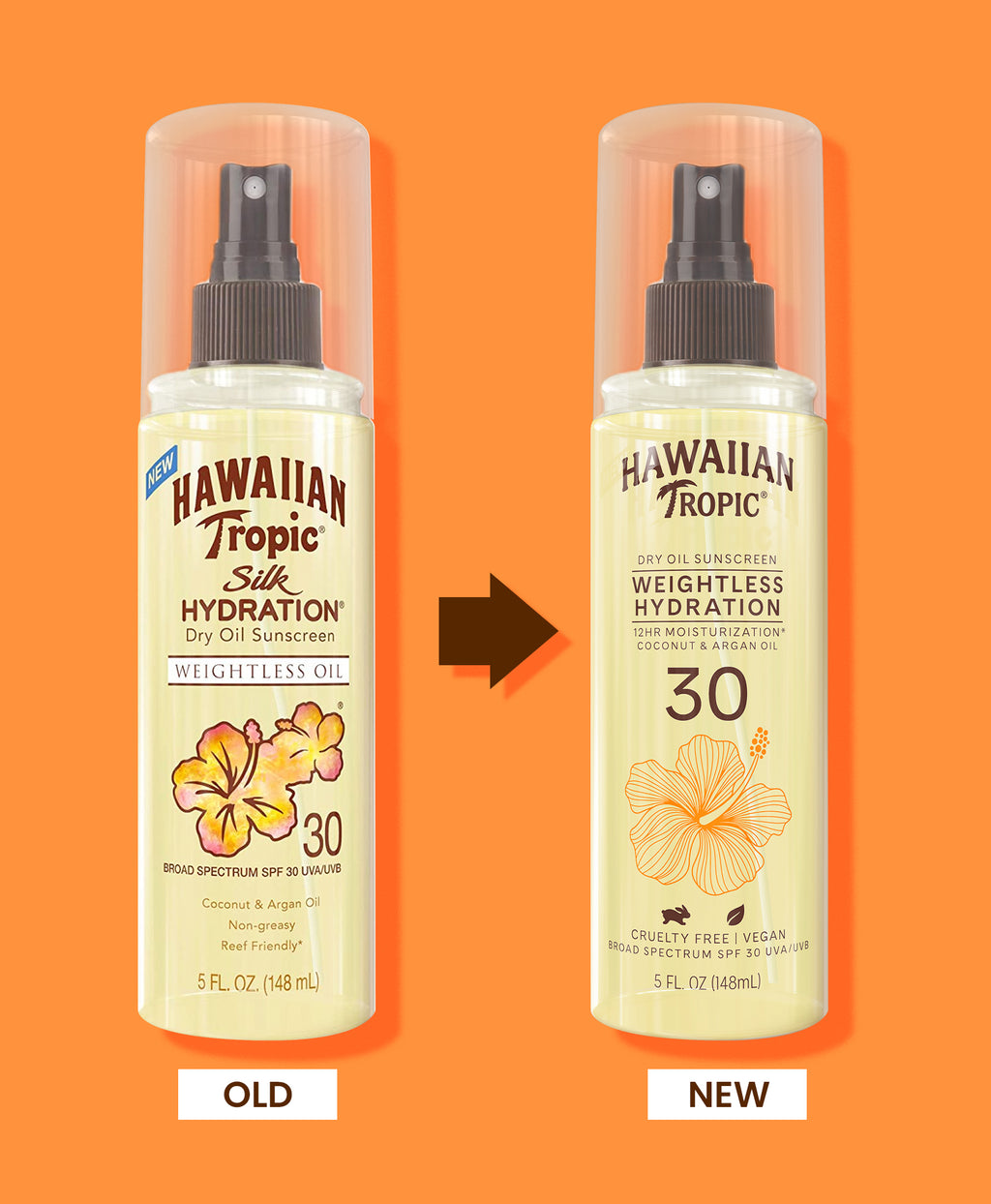The image, likely an advertisement, showcases a comparison between the old and new versions of Hawaiian Tropic Dry Oil Sunscreen. On the left, the old version of the product is labeled "Hawaiian Tropic Silk Hydration Dry Oil Sunscreen SPF 30" and features a bolder, busier design with larger logos and text. The spray bottle is light yellow with a hibiscus flower graphic and is topped with a black spray nozzle covered by a clear protective dome. The new version, displayed on the right, is called "Hawaiian Tropic Dry Oil Sunscreen Weightless Hydration SPF 30," and its design is more elegant and less cluttered, featuring a more intricate hibiscus flower graphic. Both bottles are identical in shape, size, and color, and contain similar information, including being cruelty-free and vegan. The comparison is set against a bright orange background with a black arrow indicating the transition from the old to the new product, and the labels "old" and "new" are placed beneath each respective bottle.